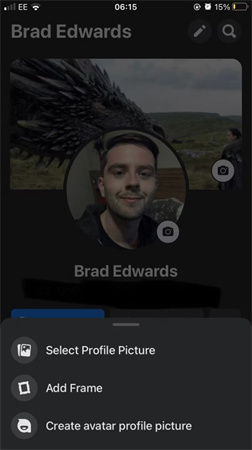The image is a screenshot taken from a cell phone, capturing a social media profile page. At the top, the name "Brad Edwards" is faintly visible. Behind this text, there is a slightly discernible background image. 

In the foreground, there is a circular profile picture featuring a man with brown hair, smiling, and wearing a black shirt. The man appears to be in his 30s. Directly under the profile picture, the name "Brad Edwards" is clearly displayed.

Two gray circles with camera icons inside are present—one overlaying the background image and the other on the profile picture. 

Near the bottom left side of the page, a blue line is visible, leading vertically beside three white icons accompanied by text. The first icon signifies "Select Profile Picture," the second indicates "Add Frame," and the third represents "Create Avatar Profile Picture." Both the icons and the text for these options are in white.